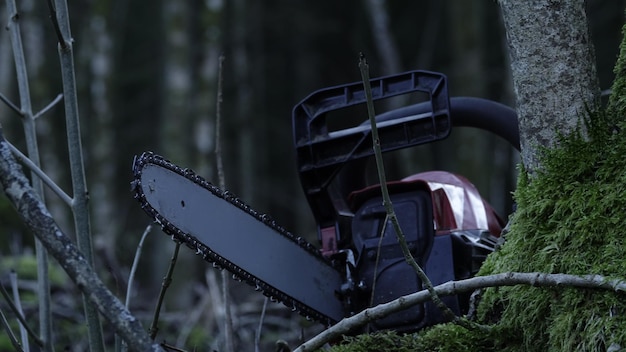A chainsaw, predominantly black with a red body and gray structural elements, is prominently featured as the focal point in this dim, blur-edged photograph. Resting unused either in the crook of a small tree or leaning against its base, the chainsaw is off, evidenced by the wood chips and debris caught in its chain. The surrounding wooded area, faintly illuminated under overcast conditions that suggest twilight or early morning, remains dark and muted, with little light penetrating the scene. Details of the environment include a tree with gray bark and a hint of green moss and small plants growing around it. The background is blurred with hints of more branches and indistinguishable undergrowth, adding to the somber, undetailed ambiance of the image.